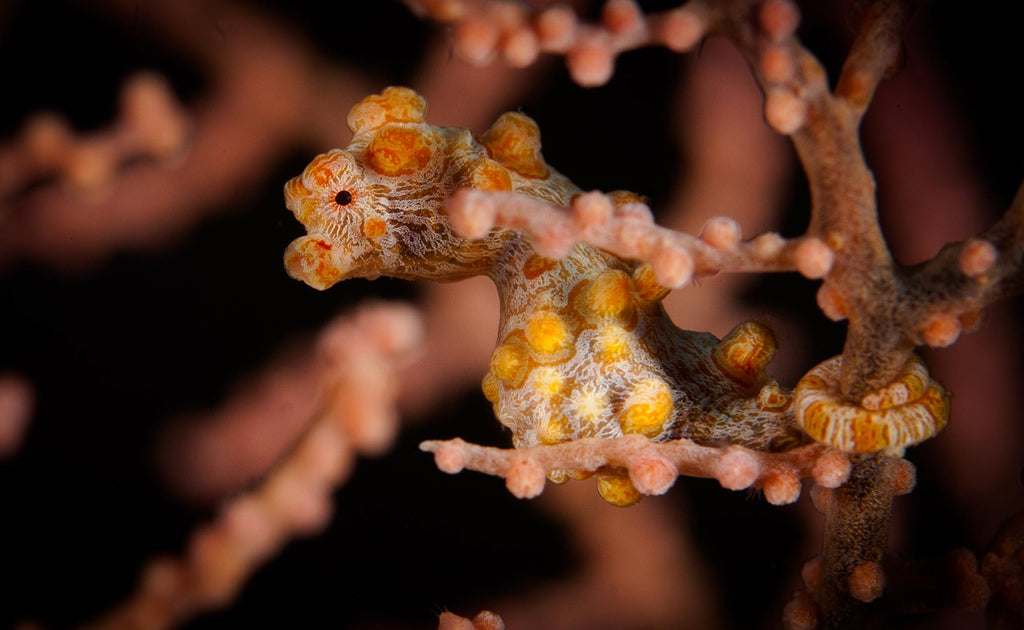This horizontally aligned photograph, possibly from a science textbook or magazine, features an ambiguous, lumpy organism that could be a type of reptile, amphibian, sea creature, or even an intricate plant. The dominant colors range from tan and peach to yellowish and reddish tones, set against a dark, blurred black background. The creature appears heavily camouflaged, blending seamlessly with its environment, which includes coral-like branches adorned with round, berry-like structures, also covered in fine white hairs.

The organism showcases a distinct texture, characterized by numerous round, circular, tumor-like bumps that are likely part of its natural structure. It appears to have a striped tail, white and yellow, that looks slightly furry and is wrapped around nearby branches. This creature has what seems to be a recognizable yellow eye and a significant round formation on its back neck, giving the impression that it is looking off to the left.

The detailed environment and the creature's intricate features make it challenging to discern whether it is an animal or a cleverly disguised plant, underscoring its role as an integral part of a complex, underwater-like ecosystem.